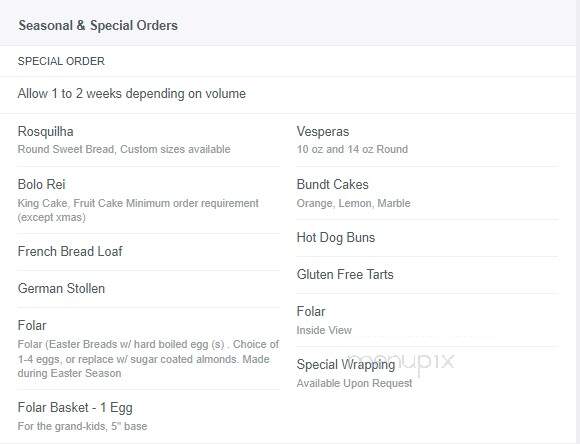This image appears to be a screenshot of a section of a website showcasing the different services it offers, specifically focusing on seasonal and special orders. The tab at the top of the section is labeled "Seasonal and Special Orders." The background is entirely white, and all the text is written in gray.

Beneath the main header, there is a sub-header that reads "Special Orders" followed by a note indicating that processing time may vary: "Allow one to two weeks, depending on volume."

The section lists various types of breads and baked goods available for order, including:
- Rose Quila
- Varespa
- Bolo Rey
- Pound Cakes
- French Roll Loaf
- Hot Dog Buns
- Gluten-Free Tarts
- Folar (repeated multiple times)
- Special wrapping available upon request
- Folar Basket, which includes one egg
- Folar, described as “Easter breads”

Behind the text, a faint watermark is vaguely visible, adding a subtle background element to the design.